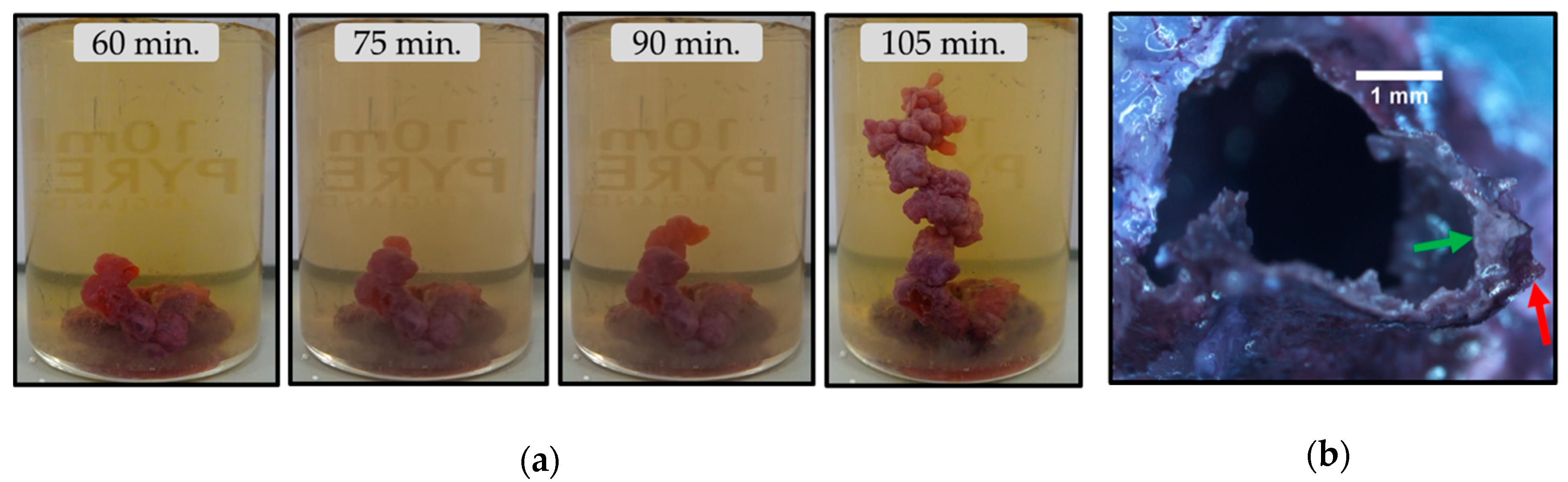**Descriptive Caption:**

This composite image series illustrates the progressive growth of a biological entity over time. The first panel, labeled "A," tracks development from a small red clump at 60 minutes, which gradually enlarges, reaching 75 minutes with noticeable growth. By 90 minutes, the clump has continued to expand, and at 105 minutes, it has grown approximately three times its initial size, evolving from a simple clump into a complex structure resembling a stalk arising from the base, composed of interconnected clumps. 

Adjacent to these images, a scale bar denoting one millimeter, accompanied by a white line, provides a size reference. The panel also includes detailed annotations: a green arrow and a red arrow point towards a specific section of a clump, marked as "B." This detailed time-lapse series underscores the dynamic and rapid growth of the entity, offering a clear visualization over a span of 45 minutes.